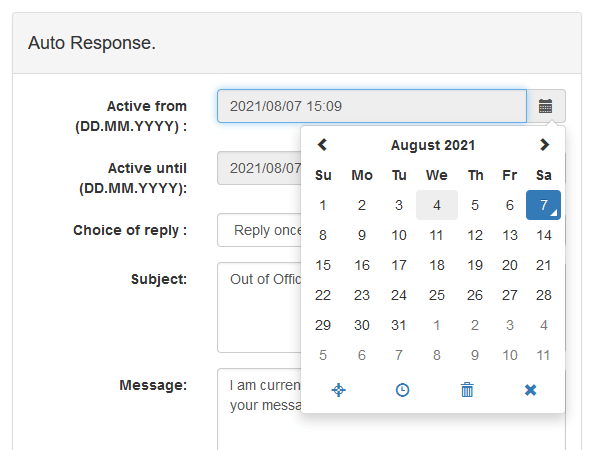Here's a cleaned up and detailed caption for the image:

---

**Screenshot Description:**

This appears to be a screenshot, possibly taken on a mobile phone, featuring a clean, predominantly white interface. The top portion of the image is distinctly marked by a thin gray pixel border, but the bottom part is cut off.

The interface seems to be related to setting up an auto-response for emails or messages. At the top, there's an input field labeled "Active from dd.mm.yyyy," where the user has entered "2021/08/07 15:09". This field has a pink background and includes a calendar icon on the right, which, when selected, displays a calendar for August 2021. The calendar view shows navigation arrows for moving between months, with the days of the week (Sunday through Saturday) formatted in bold at the top, and daily dates listed below, starting with Sunday the 1st. The calendar also incorporates dates from the following month, September, in gray, extending down to Saturday the 11th.

Below this, there are four blue icons arranged from right to left: a close button, a trash can icon, a time setting icon, and a map icon, all representing different functionalities.

Underneath the "Active from" field, there’s another input labeled "Active until," containing the same date within a similarly styled pink field. However, this part is obscured, so the exact time isn't visible.

The following section includes settings for the auto-response message, with options such as "Choice of reply: Reply once," the subject "Out of Office," and the beginning of a message content that starts with "I am currently..." but is cut off beyond that point.

Overall, the screenshot provides a visual overview of configuring an auto-response, highlighting calendar integration and various setting options.

---